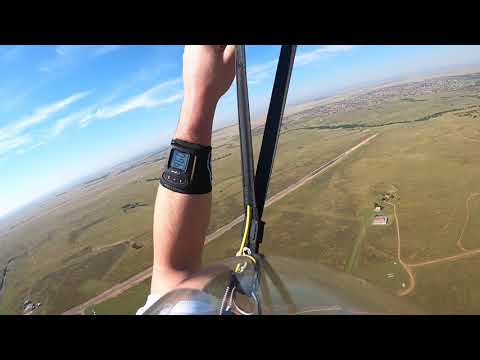This is a photograph captured from a GoPro, likely during a skydiving or parachuting activity, featuring a white person's outstretched arm adorned with a black wristband displaying numbers. The arm extends vertically, and you can observe ropes or tethers connecting to carabiners, which go out of the frame, hinting at the parachute above. The background reveals a panoramic aerial view of the rural countryside below, characterized by brownish-green fields, a sparse population, and a prominent dirt road. The earth’s curvature is subtly visible, with the blue sky and clouds enhancing the expansive scene. The image, though of lower quality, vividly conveys the exhilarating perspective of high-altitude flight.